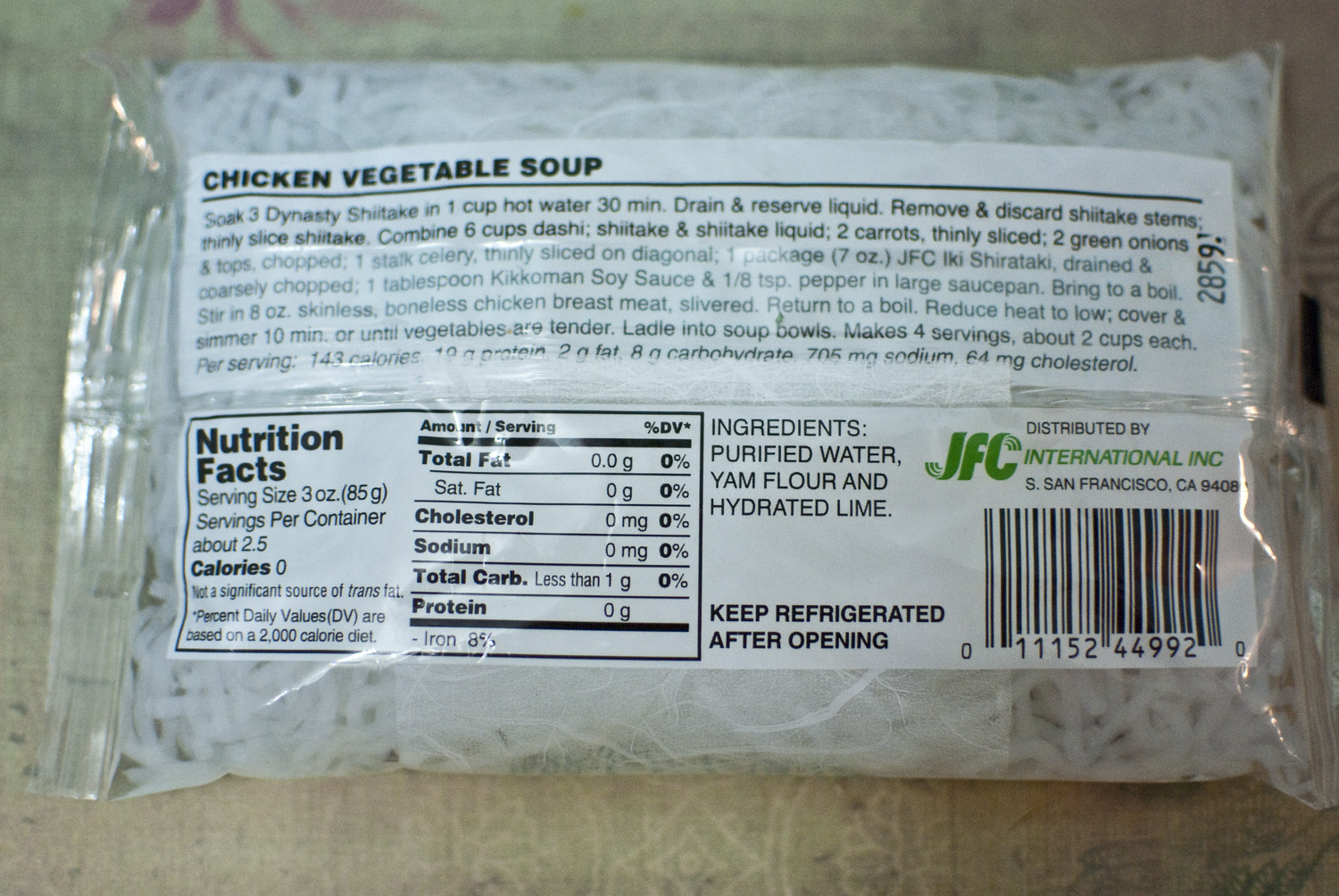This photograph displays the back of a food package wrapped in clear cellophane, revealing thin white noodles inside. The background of the package features a beige color with accents of red and green. Prominently in the center is a large white rectangular area. In the upper left corner of this rectangle, the words "CHICKEN VEGETABLE SOUP" are boldly printed in black, all-caps font. Beneath this title, a paragraph of black text provides additional information.

A white horizontal strip runs across the middle section of the package. On the lower left side of this strip, there is a horizontal rectangle labeled "Nutrition Facts." Directly to the right of this, the ingredients are listed at the top, followed by the phrase "Keep refrigerated after opening."

At the top right corner, "JFC International Inc." is printed in green, with the phrase "Distributed by" and more information in black text directly below it. Located in the lower right-hand corner is the barcode, completing the informative layout of this food package.